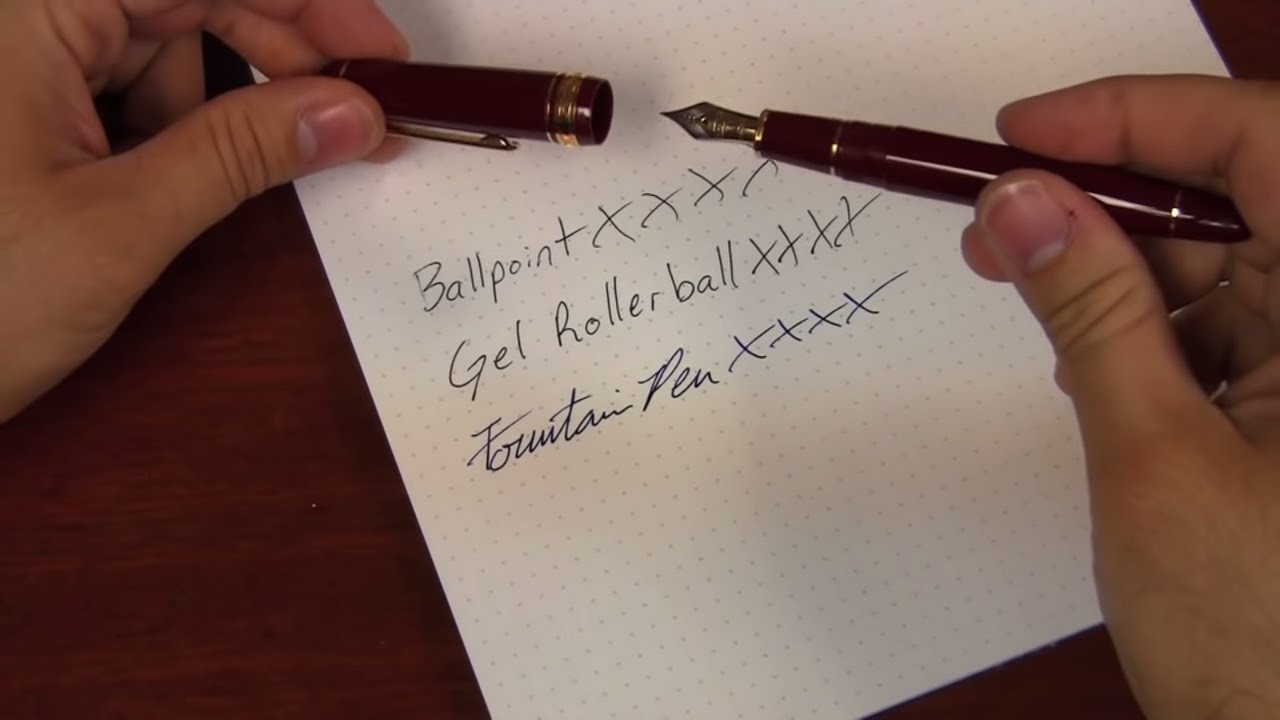In this indoor photograph, we're looking down from the perspective of someone writing. The image is rectangular, about five inches wide and three to four inches high, depicting a wooden tabletop with a white piece of paper on it. The paper, adorned with light gray dots for guidance, is slightly angled. Three sections of handwritten text are visible on the paper: the first reads "ballpoint" followed by four X's, the second says "gel rollerball" with another set of four X's, and the third is "fountain pen" written in blue ink, again with four X's.

Above the paper, a pair of hands, likely feminine with light brown skin, is seen holding a fountain pen. The right hand grips the pen's barrel, which is dark red with a brownish hue, featuring a fine, pointed tip reminiscent of antique pens. The pen has two gold bands around the barrel, and the cap, held in the left hand, has additional gold bands and a clip. The wooden surface of the desk frames the hands and paper, grounding the scene in a natural, warm-toned setting.